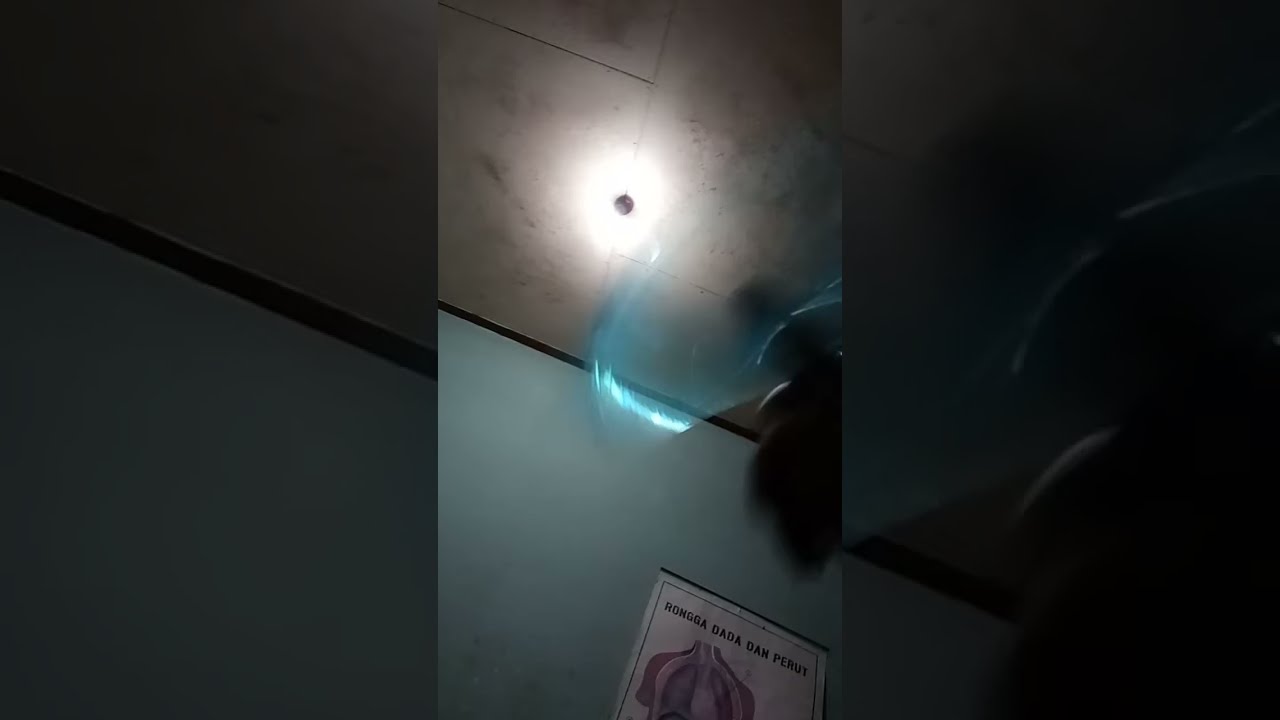The photograph captures the silhouette of a black hand, prominently positioned against a bright, light-filled background, creating the impression of an x-ray due to the lighting. The hand is centered on a sleek, high-definition screen that resembles a white desk adorned with additional items, such as a pencil and two pads—possibly prescription pads—that are partially cut off at the edges. This central image, shaped like a smartphone, is flanked by faded-out, semi-transparent sections of the same image, both on the left and right sides. The left side features a faded portion of the x-ray screen, while the right side shows a blurred section of the silhouetted hand. In the background, you can see white walls with tan ceiling tiles and light pink flyers scattered about. A bluish-white arc or swirl of light appears around the finger, adding a dynamic, swirling motion to the scene. The overall effect is that of a hand casting its shadow against a brightly illuminated space, blending both clarity and abstraction.